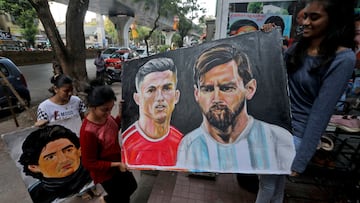In this horizontally-aligned, rectangular photograph, likely taken in South or Southeast Asia, several young women with dark hair and tan skin are gathered on a brick stairway, a sidewalk visible to the side, and a street with parked and driving cars bordered by trees and a brick wall in the background. The central focus is on two women holding a detailed rectangular painting of two men. 

The man on the left in the painting has a somewhat annoyed or concentrated expression, with his dark hair combed back and shaved on the sides, a small goatee, and is wearing a red shirt with white shoulder stripes. He appears to be around 30 years old. The man on the right, likely about 40, has a beard and mustache, dark brown hair parted on the right, and is wearing a pale light purple and blue striped shirt. Both men’s torsos face slightly to different directions while their faces are turned towards the front. 

The painting is held by a woman in a red long-sleeved top and black pants on the left, who looks down with her hair tied back, and another woman in a blue long-sleeved top on the right, appearing to smile. To their left, another woman in white with dark-checked sleeves holds a square painting of a man with a feathered 70s-style black hairstyle, dressed in a black turtleneck against a gray background. 

The scene is set outdoors during the daytime on a busy street, capturing not only the women and their paintings but also the bustling urban environment around them.